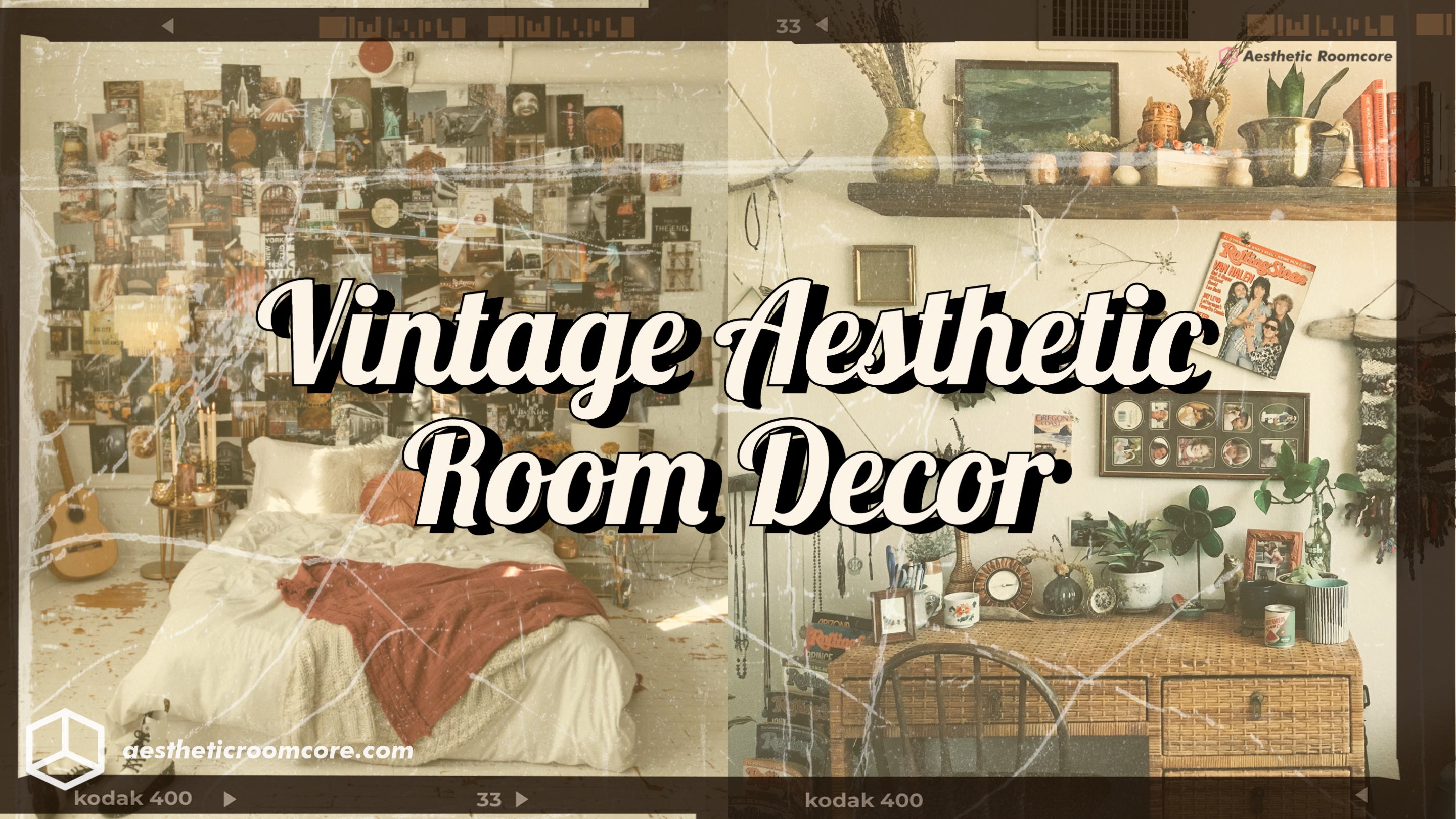In this image that has a strong old-time advertisement vibe, the text "Vintage Aesthetic Room Decor" is prominently displayed in the center with a retro, funky font. The white letters, accented with a thin black outline and a bold black drop shadow, give the text a striking presence. The image is framed by a dark brown photo negative-style border, adding to its vintage appeal.

The background features two distinct pictures. On the left, a cozy bedroom is shown with a white comforter and red blanket atop a bed surrounded by white pillows. The entire wall behind the bed is covered in various posters, including a Rolling Stone magazine cover, adding a nostalgic touch. A guitar rests to the left of the bed, enhancing the room's retro ambiance.

On the right side, a brown desk, cluttered with assorted objects like plants, a mug, and possibly a picture, comes into view. Above the desk, the wall is adorned with frames and a shelf near the ceiling holding various items. The room elements and decor, combined with the film filter and aged look of the walls, convey a sense of historical charm. Additionally, there's a watermark on the lower left side that reads "aestheticroomcore.com."